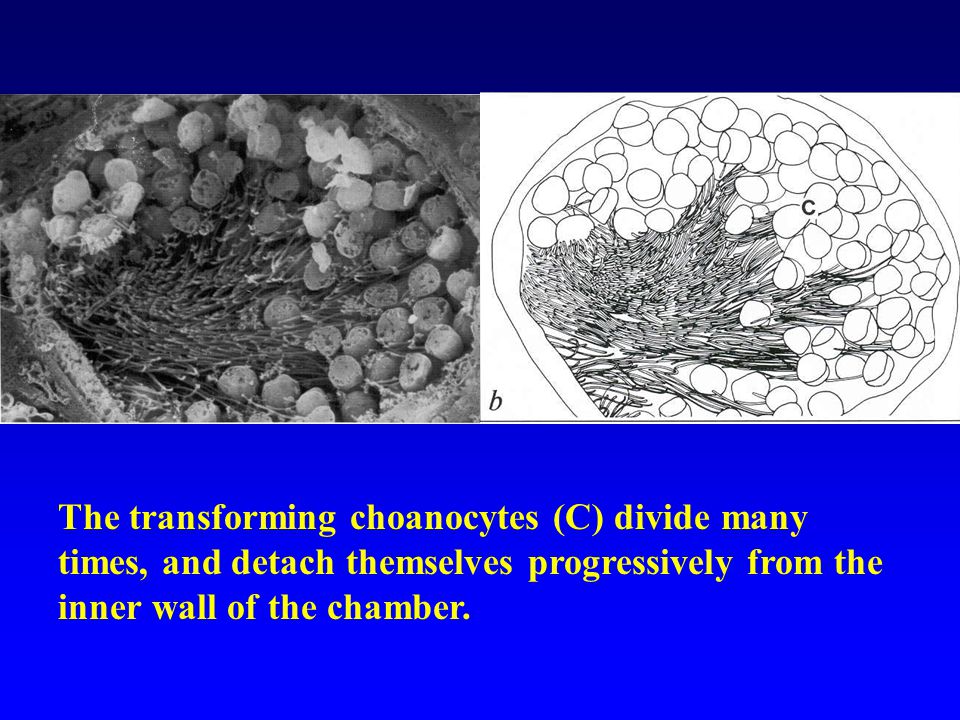The image appears to be a slide from a PowerPoint presentation or a textbook, featuring a structured and detailed visual explanation. The upper portion of the slide displays a dark deep blue banner while the lower section has an almost neon, very bright blue box. Within this box, yellow font text reads: "The transforming choanocytes (C) divide many times and detach themselves progressively from the inner wall of the chamber." 

On the left side of the image, there is a black and white photograph showing a close-up view of choanocytes, with distinct features that resemble tiny, string-like structures. To the right, there is a corresponding black and white drawing of a choanocyte, highlighting the same details but in a more schematic form. This drawing includes a letter "B" in the bottom left corner and a letter "C" within the cell depiction. The overall design suggests an educational context, illustrating the morphological changes and behavior of choanocytes.